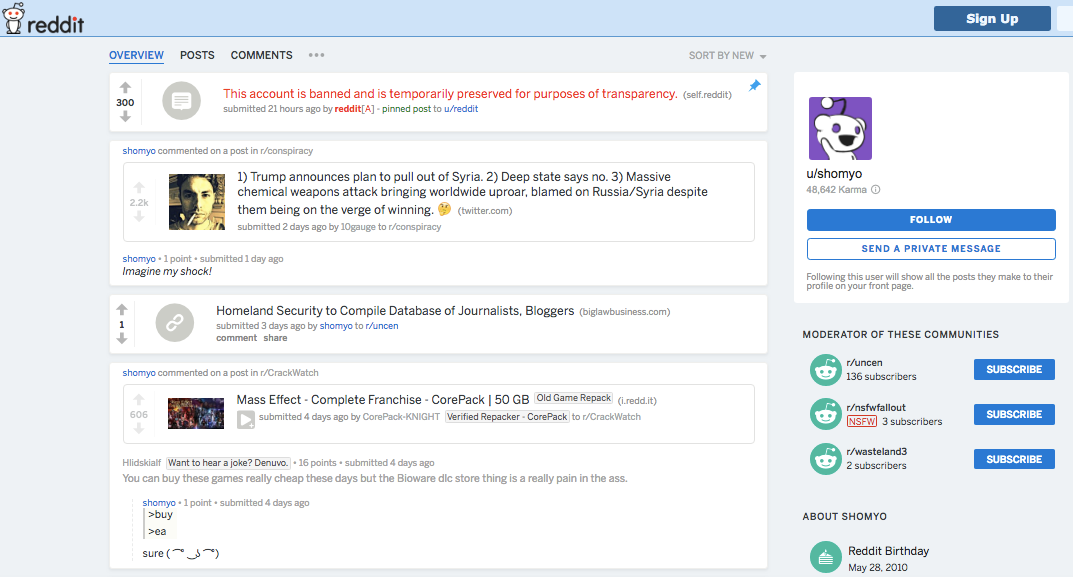This image is a cropped screenshot of a Reddit webpage featuring a light blue header and an even lighter blue background. In the top left corner, the Reddit logo is displayed alongside the word "reddit" in black letters. To the far right of the header, there is a prominent blue "Sign Up" button.

Below the header, the body of the webpage consists of user interface elements and posts. Positioned at the top left within the body are three options: "Overview," "Posts," and "Comments." The "Overview" tab is selected and highlighted in blue, with a blue line underneath it, indicating it is the active section.

The main content area features posts displayed within white boxes. The top post contains a message stating, "This account is banned and is temporarily preserved for purposes of transparency," written in red text. To the left of this message is a gray icon featuring a chat bubble. Adjacent to the icon, towards the right, are upvote and downvote arrows with the number "300" between them, indicating the post has been upvoted 300 times.

Below the top post, another post follows the same format. The arrangement includes the upvote and downvote arrows on the left, with the number of upvotes displayed in the center. To the right of the arrows, there is a profile picture, followed by the text of the post to its right.